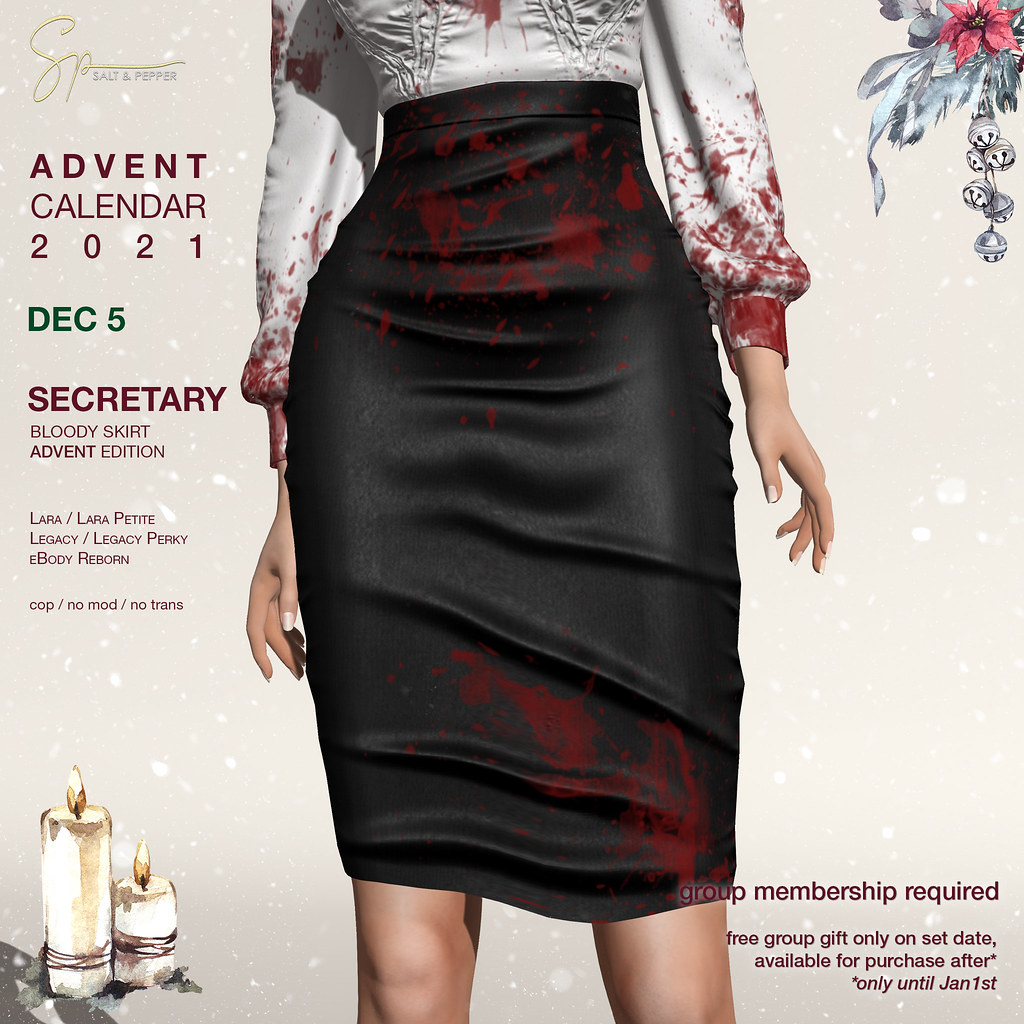This image is an ad for a clothing item featured as part of the Salt & Pepper Advent Calendar 2021. The ad prominently displays the date December 5 and promotes the "Secretary Bloody Skirt Advent Edition." The featured clothing includes a black skirt splattered with what appears to be red blood or paint, and a long-sleeved red and white shirt with similar red splatters. The model shown in the image is only visible from just below the breasts to the knees. The upper right corner of the ad showcases a poinsettia-like holiday flower, greenish-white with pink shading, and accompanied by six jingle bells. In the bottom left corner, there are two lit white candles. The ad notes that the outfit is compatible with multiple body types including Lara, Lara Petite, Legacy, Legacy Perky, and eBody Reborn, and specifies that it is COP/no MOD/no TRANS. Additionally, it mentions that group membership is required for a free group gift on the set date, with the item being available for purchase until January 1st.